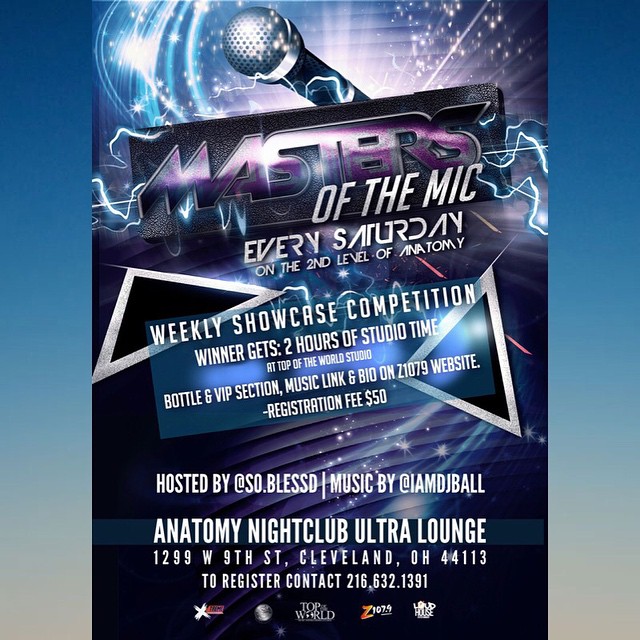Introducing "Masters of the Mic," an exhilarating weekly showcase competition held every Sunday at the Anatomy Nightclub Ultra Lounge, situated at 1299 West 9th Street, Cleveland, Ohio. This electrifying event offers budding artists a chance to shine, with the winner earning two hours of studio time at Top of the World Studio, a bottle and VIP section, and a coveted music link and bio on the Z1079 website. 

Regarded for its vibrant visuals, the advertisement for this event features a dazzling design set against a blue and black gradient background, highlighted by whitish blue sparkles, electricity, and streaks of light. At the center, a microphone emits a radiant glow, surrounded by purple and blue hues. The bold title, "Masters of the Mic," is prominently displayed in striking white and purple text, accentuated by lightning-like edges. Further details about the competition are provided in white text, mentioning the $50 registration fee.

Hosted by the charismatic @so.blessed (spelled B-L-E-S-S-D with one E) and featuring music by the talented @iamdjball, this event promises an unforgettable night of music and entertainment. The detailed graphics include thin white strips resembling blinds in the background, adding an artistic touch to the overall composition. Don't miss out on this incredible opportunity to witness or compete among the best talents every Sunday night.